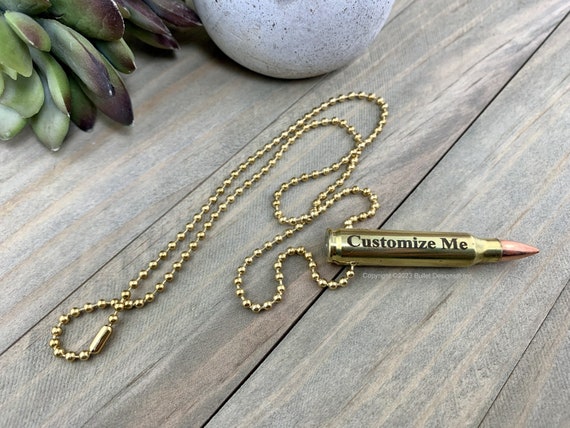In the image, there is a small, golden, shiny object with black text that reads "Customize Me." The object resembles either a pen or a lipstick, with a peach-colored tip that adds to the ambiguity—it could be a drawing instrument or a cosmetic item. It is attached to a gold chain made of small, round balls, typical of the kinds used to prevent loss. The chain threads through the device, with one end coming out the other side, and it weaves around, extending towards the bottom left of the image.

In the upper left corner, the picture includes some green and gray objects that might be succulents, feathers, or vegetables, casting a natural element into the scene. Centrally, at the top margin, there is a partial view of a white, globe-shaped object speckled with various colors, possibly a concrete planter. All these items rest on a weathered wooden surface, displaying distinct brown, gray, and tan planks arranged diagonally from the top right to the bottom left. The overall coloration and texture contrast with the metallic and shiny appearance of the central object, enhancing its prominence.